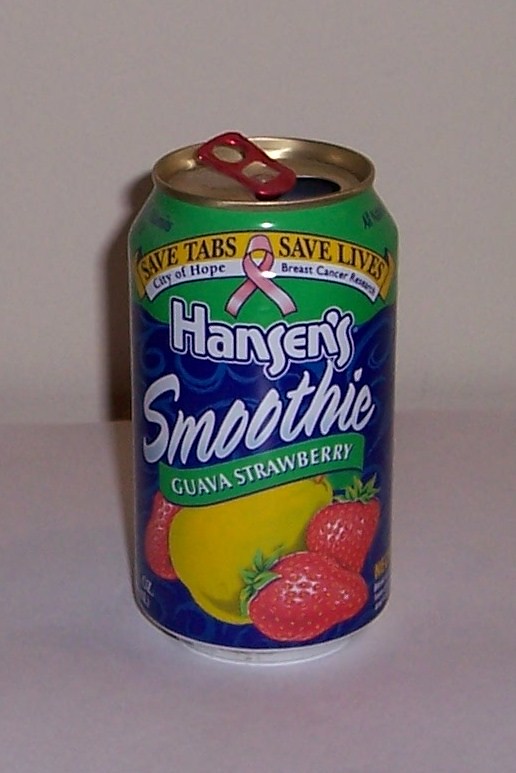This image features a 12-ounce aluminum can of Hansen's Smoothie Guava Strawberry. The can has a golden top with a bright red pull tab, and it is open. The upper part of the can is green, transitioning to a blue background with lighter blue swirls down the body. A yellow and white banner near the top reads "Save Tabs, Save Lives" and prominently features a pink breast cancer ribbon with text underneath that says "City of Hope Breast Cancer Research." The main white text "Hansen's Smoothie" is displayed across the blue portion of the can, while a green banner at the bottom contains the words "Guava Strawberry" in white text with a blue outline. The label also showcases images of three pink strawberries with green tops surrounding a central guava. The can is positioned on a very light mauve-colored countertop with a whitish wall in the background. Some additional writing is present on the side of the can, but it is not fully visible from the current angle.